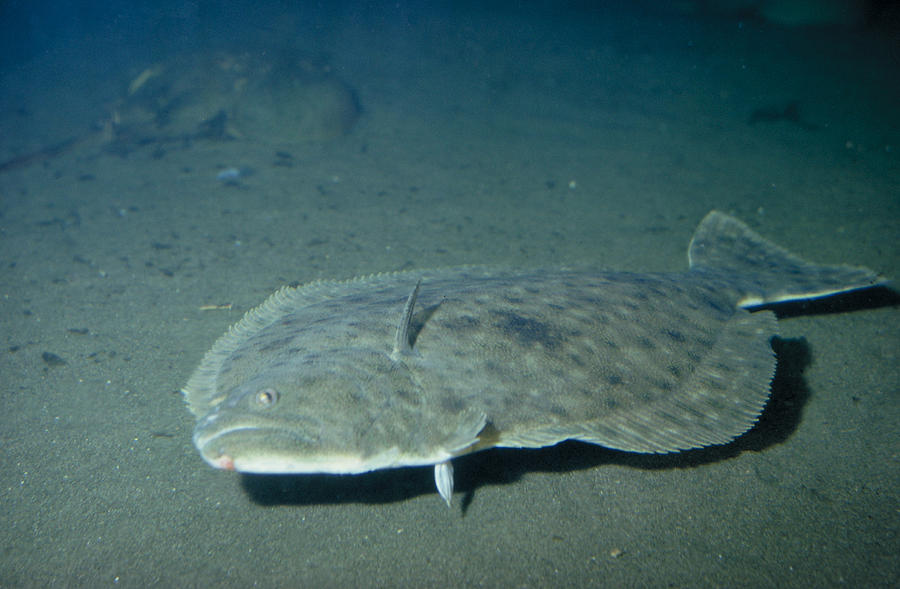The image depicts a very large, flat fish lying horizontally on its side at the bottom of the ocean. The fish, which has a grumpy or downturned mouth, blends seamlessly with the sandy, compressed seafloor due to its grayish-green, mottled coloration with some black spots predominantly along its upper side. It has two small flippers protruding from its sides, a distinct ridge running along its back, and spines on both its top and bottom. The fish’s tail is broad and flat. Intriguingly, it is positioned in a way that one of its eyes faces the ground, adding to its unusual appearance. The surrounding area features a rock in the upper right corner and some small black rocks scattered between the fish and the larger rock. The top part of the image fades into a darker brown hue, giving the scene a slightly eerie ambiance.